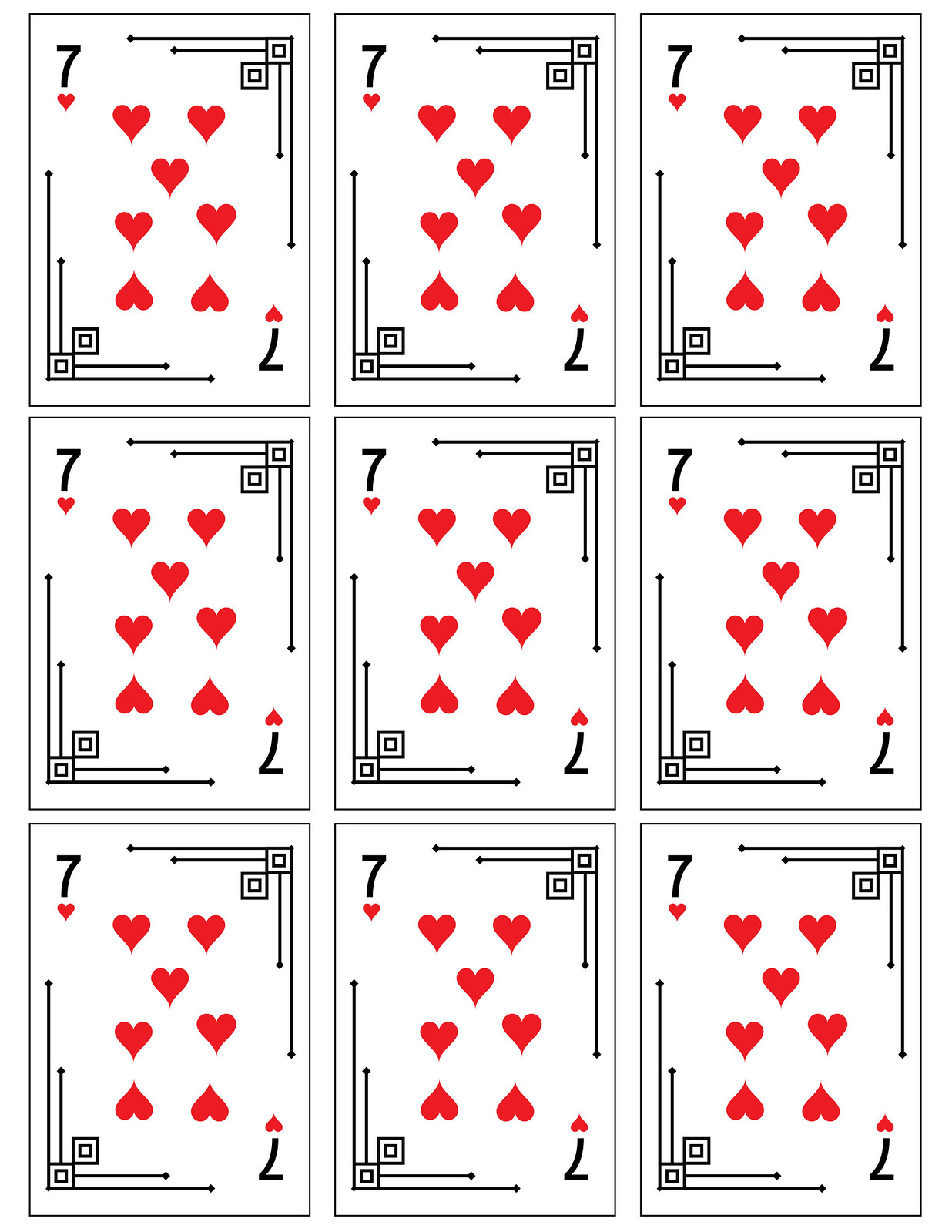This image is a detailed drawing set in portrait mode, showcasing a grid layout composed of three rows and three columns, totaling nine identical cards. Each card is the seven of hearts, meticulously depicted with classic design elements. 

On each card, the upper-left corner features a red number "7" above a small red heart, while the bottom-right corner displays an inverted red "7" and an inverted heart, which is typical for playing cards. Each card also features seven red hearts arranged in a symmetrical pattern within the center.

The background design of each card includes a decorative motif: two black squares positioned centrally, with thin black arrows extending outward in each cardinal direction—up, down, left, and right.

This organized array of nine seven of hearts cards creates a visually striking composition. The repetition and precise arrangement provide a sense of modern art or conceptual design, making a bold statement with its symmetry and simplicity.